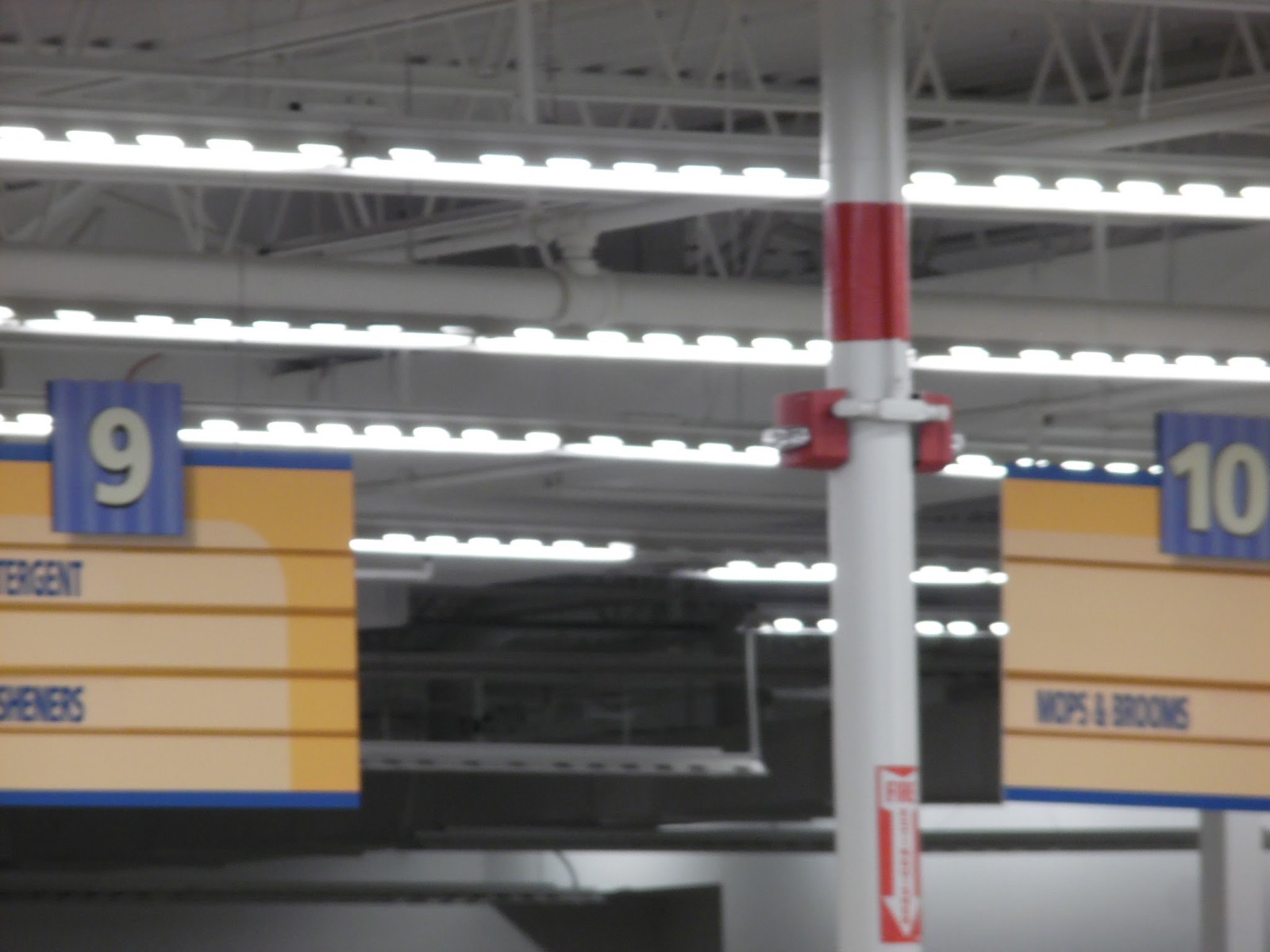The photograph captures the interior of a large, austere warehouse store, focusing on its ceiling and upper infrastructure. The ceiling is constructed of a metal roof supported by steel trusses, each triangular truss bottom adorned with fluorescent lights. The slightly blurred lighting creates the illusion of four horizontal lines traversing the image. Prominent white pipes and columns are visible throughout the space.

Two rectangular aisle marker signs are discernible: one labeled "9" and the other "10." Aisle 10 features mops and brooms, while Aisle 9 likely stocks detergent and air fresheners. The signs have a yellow background for the descriptions of aisle contents, and the aisle numbers are displayed in white letters on blue squares. Centrally positioned is a column marked with a fire extinguisher sign and accompanied by various red fire alarm components, adding a touch of color to the otherwise stark environment.